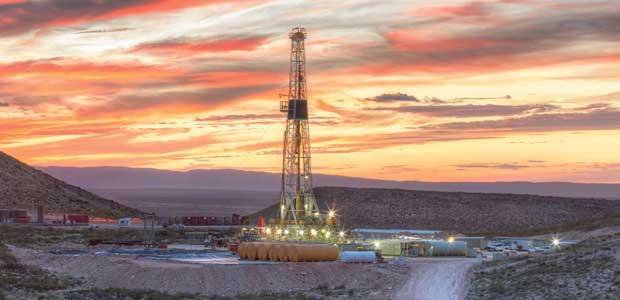The photograph captures a desolate oil drilling site against a dramatic tangerine sky, likely taken at sunset. The scene showcases an oil rig, enveloped in bright yellow lighting at its base, with intricate metal scaffolding around it. The landscape is predominantly flat with a few hills and an outline of extreme mountain ranges fading into the misty background. Scattered across the dirt ground near the rig are several large brown cylinders, reminiscent of tanker tanks, and various storage containers, pipes, and drums. The evening light casts a warm yellow glow on a cluster of gray buildings situated to the right of the drill, while a dirt road winds through the barren landscape, past the equipment and buildings. The sky, a rich tapestry of purples, golds, umbers, oranges, reds, whites, and grays, adds a melancholic beauty to the otherwise stark and industrial scene.